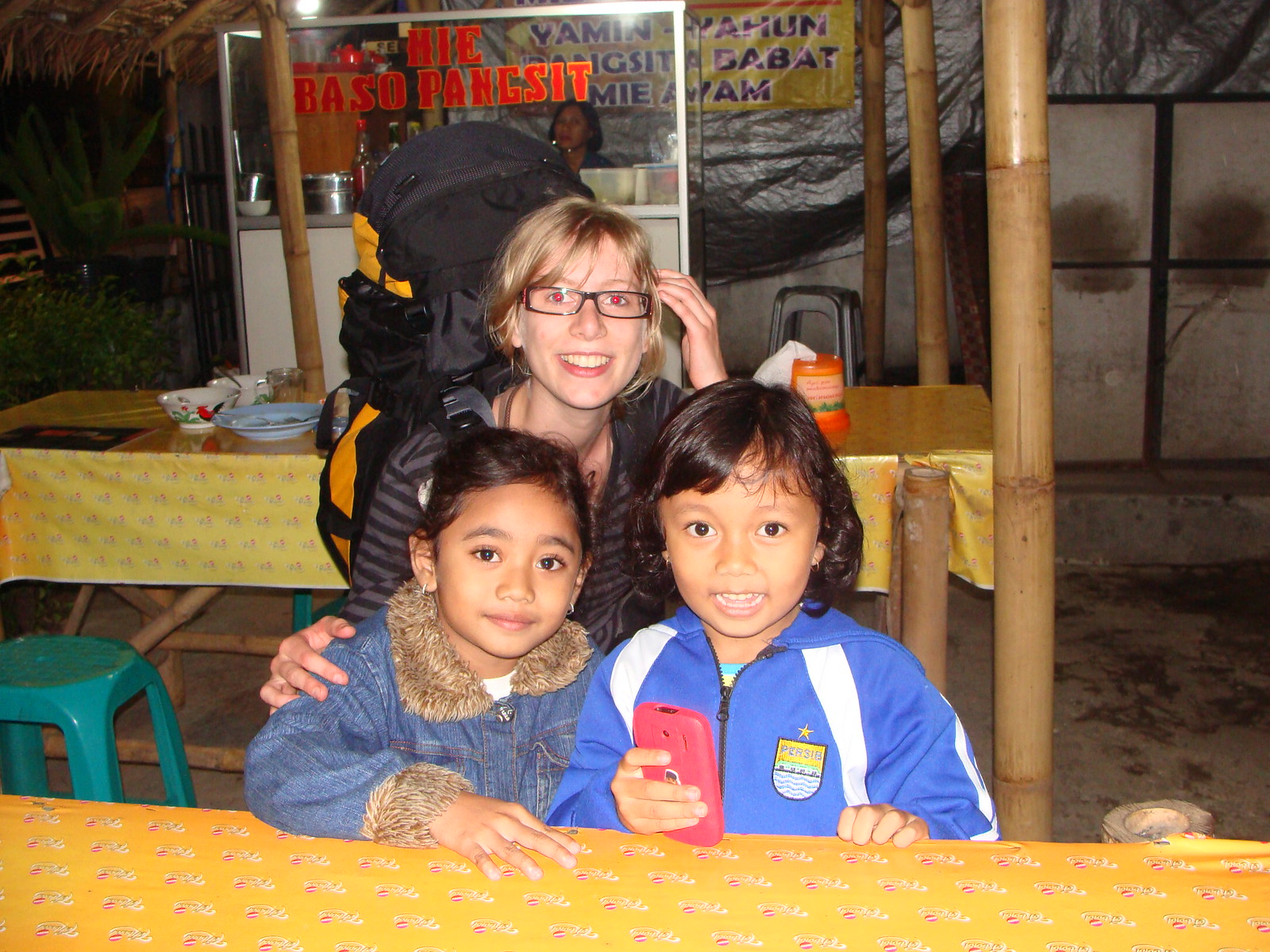The image captures a nighttime scene in an outdoor setting that resembles a primitive village or a rustic restaurant. The photograph is rectangular and taken in a hut-like structure, supported by bamboo beams with a grassy roof. In the background, a stand with pots and pans suggests a cooking or serving area. Several tables with yellow plastic tablecloths are seen, adding a vibrant touch to the otherwise subdued environment. On the left-hand side, a counter is partially closed off, with a lady who appears to be a cook standing behind it.

At the center of the image is a young woman with short blonde hair, wearing black-rimmed glasses and a large black and yellow backpack, indicative of someone who is possibly backpacking or traveling. She is seated at a table with two young girls. The girl on the left, with dark hair pulled back and small earrings, wears a jean jacket with fur trim on the collar and cuffs. The girl on the right sports a blue and white tracksuit jacket and holds a pink cell phone. Both girls are smiling at the camera, capturing a moment of cheerfulness.

Additional details include a teal aqua chair or stool on the left side of the frame and some text in red on a clear glass screen in the background, possibly written in a different language. The overall atmosphere suggests a communal or village setting where the woman appears to be a visitor, engaging with the local children.